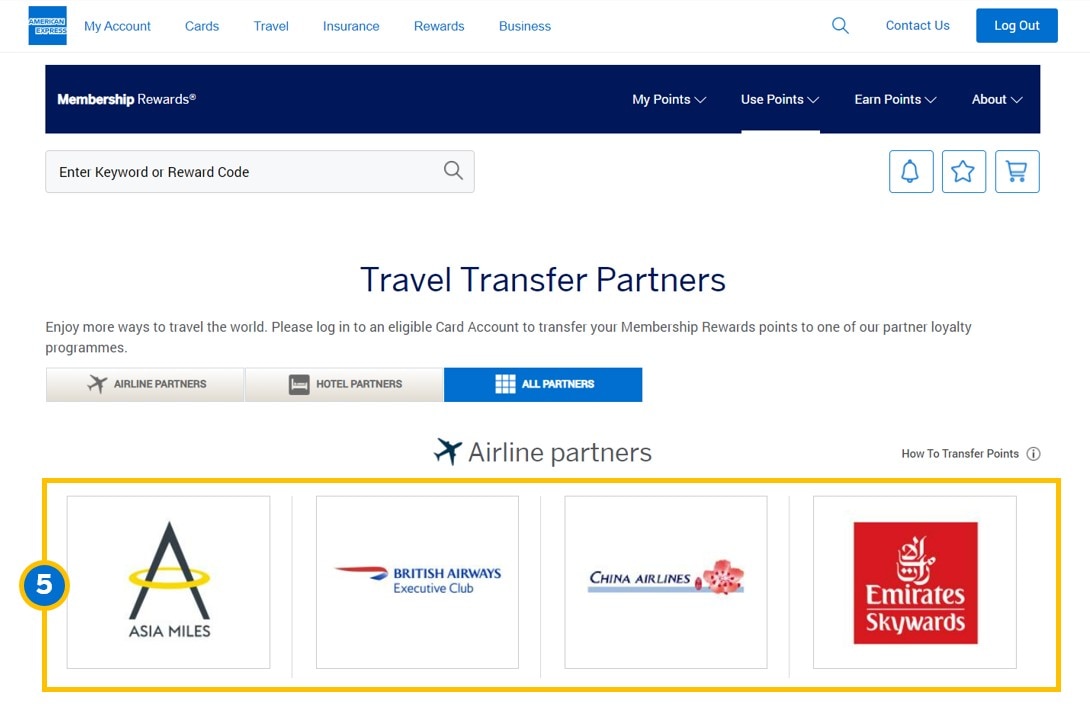**Image Description:**

On a white background, the image features components related to the American Express website interface. At the top, there is a navigation menu containing options such as "My Account," "Cards," "Travel Insurance," "Rewards," "Business," and a blue magnifying glass symbolizing the search function. Additional links include "Contact Us" and "Log Out." 

Below the navigation menu, there is a prominent blue rectangle with white text that reads "Membership Rewards." Underneath this, there is another menu with options like "My Points," (which is underlined), "Use Points," "Earn Points," and "About."

A search bar is prominently displayed with the placeholder text "Enter keyword or reward code," accompanied by a magnifying glass icon. To its right, there are icons for a notification bell featuring a star and a shopping cart.

The main body of the image presents a message about travel transfer partners: "Enjoy more ways to travel the world. Please log into an eligible card account to transfer your Membership Rewards points to one of your partner loyalty programs." Below this message are three rectangles (two gray and one blue) providing categories for transfer options: "Airline Partners," "Hotel Partners," and "All Partners." 

Under "Airline Partners," there is information on "How to Transfer Points." A rectangle surrounds four squares, each containing the names and icons of different partner airlines. A blue circle with a white number five is present, indicating five options: "Asia Miles," "British Airways Executive Club," "China Airlines," and "Emirates Skywards."